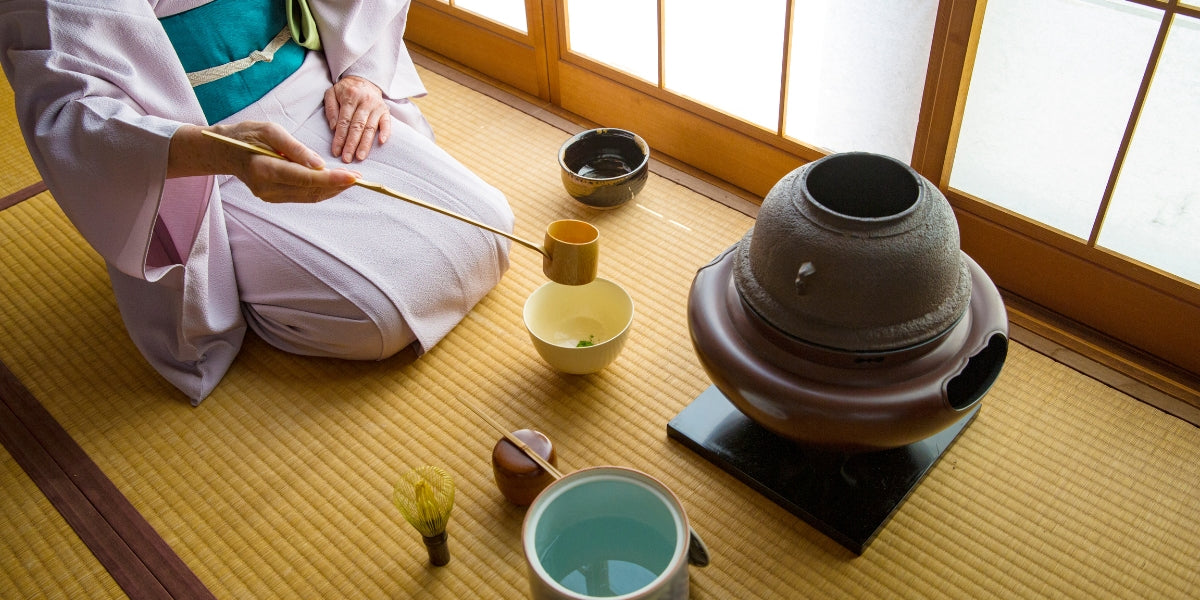In this photograph of a Japanese tea ceremony staged inside a traditional Japanese-style room, a woman is preparing tea. The room features light brown floor coverings and sliding rice paper doors with frosted glass and light wooden frames. The woman, positioned on the upper left, is kneeling on what appears to be a straw mat or rug. She is dressed in a pink kimono with a teal blue front. Her face is cropped out of the frame, but her actions are clear: she holds a long-handled bamboo ladle, pouring water into a yellowish bowl in front of her. In the center foreground is a large brown pot with either a metal or clay top. Various traditional tea accessories are arranged around her, including a smaller brown bowl to her left, a white pot with a pink exterior to the right, a brown container with chopsticks on top, and a bamboo tea whisk or frother. The careful arrangement and traditional elements captured in the image suggest a serene and culturally rich scene of a Japanese tea ceremony.